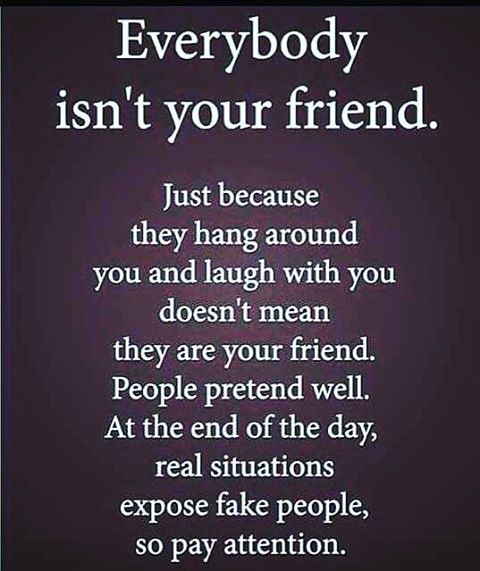The image features a predominantly dark plum purple background, which lightens towards the center in a soft gradient. The text is prominently displayed in a centered alignment and is written in white. The message reads: "Everybody isn't your friend. Just because they hang around you and laugh with you doesn't mean they are your friend. People pretend well. At the end of the day, real situations expose fake people, so pay attention." The quote spans nearly the entire vertical length of the rectangular image, emphasizing the importance of discerning genuine relationships in real situations.